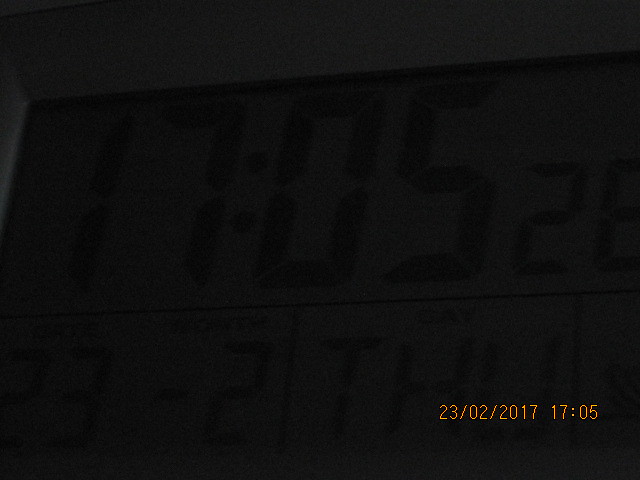The image appears to be a very dim photograph with a dark gray to nearly black background. In the bottom right corner, there's a timestamp in orange numbers reading "23/02/2017, 1705." The time "1705" is also prominently displayed in large, dark figures near the center of the image. The bottom left corner contains vague lettering that might include "33-2" and potentially the word "Thursday." The rest of the image is indistinct and largely blacked out, making it difficult to discern further details. The overall impression is of a clock or similar display in a very dark setting, with blurred and obscured elements that challenge visibility.